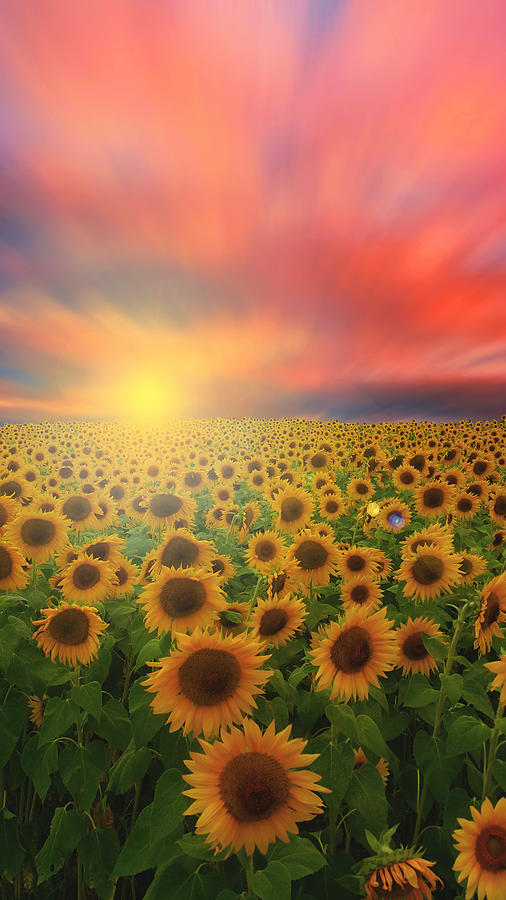The image presents a vast, mesmerizing field of mature sunflowers stretching endlessly to the horizon under a heavily edited sky. Each sunflower, towering and vibrant, boasts several pointed yellow petals encircling a large dark brown center, all perched on sturdy green stems with multiple pointed leaves. Unnaturally, all the sunflowers face directly towards the viewer, rather than the sun setting towards the center left of the image. The surreal sky above features a visually striking gradient of pink, orange, and red tones with dark blue splotches and clouds that seem to rush upward, despite the still nature of the photograph. The visually dramatic sun, glowing yellow, contributes to the ethereal and almost fantastical ambiance of the scene. This digitally enhanced sunset, coupled with the unique orientation of the sunflowers, creates a captivating and surreal visual experience.